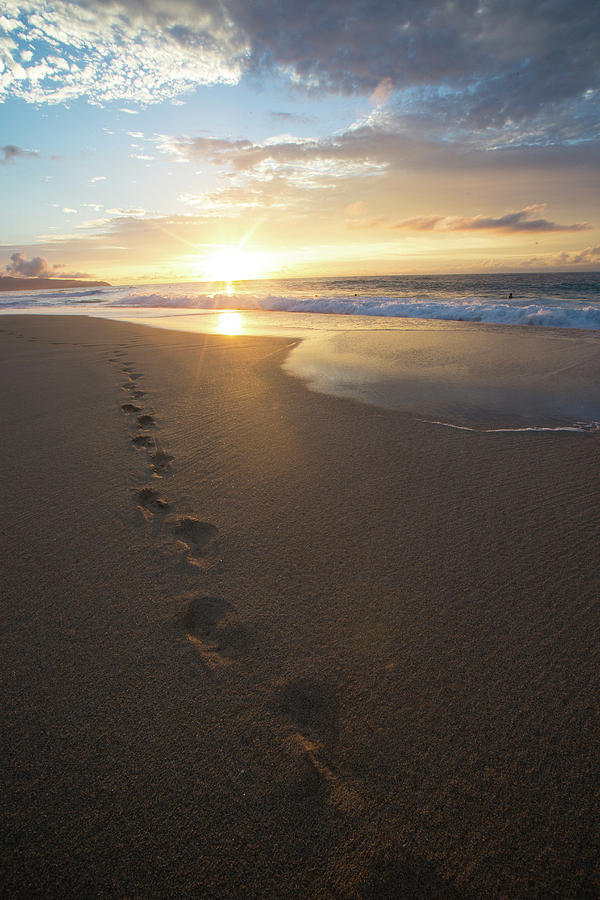In this vertically aligned rectangular photograph, an enchanting beach scene unfolds during early evening. The serene setting sun hovers just above the water in the image's upper middle portion, casting a radiant yellow glow and illuminating the sky with hues of yellowish-brown. The sky is a stunning blend of colors, showcasing clear blue tones on the left, mingling with pretty white feathery clouds in the upper left corner, and transitioning to gray feathery clouds in the upper right. Below the vibrant sky, a large wave hits the shoreline, its white foam contrasting against the grayish backdrop of the water.

The foreground features packed sand, dark brown in color, with a series of footprints meandering from the lower right side towards the left, leading towards the water. The sun's brilliant rays bathe the shallow, gentle waves in a warm light, enhancing the overall beauty of the tranquil seashore. There are no other people present, making the beach appear peaceful and unspoiled, capturing a perfect, fleeting moment of natural splendor.